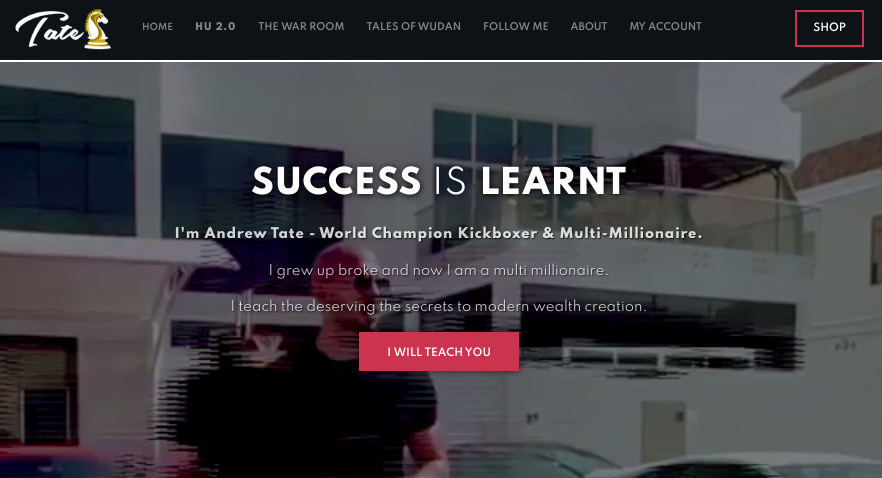This is a detailed caption describing a screenshot of Andrew Tate's website:

---

The screenshot captures the top section of Andrew Tate's website. Dominating the header is a sleek black banner featuring Andrew Tate's logo on the left, a stylized chess piece, with his name displayed prominently to the right. The website's navigation menu spans across the top, listing categories such as Home, HU 2.0, The War Room, Tales of Wudan, Follow Me, About My Account, and Shop. A red box highlights the 'Shop' category, indicating a call to action to explore this section.

Beneath the navigation bar, a striking background image forms the canvas for an overlay of bold typography. The potent phrase "SUCCESS IS LEARNT" is prominently displayed with 'Success' and 'Learnt' in bold. Below this, a personal introduction reads: "I'm Andrew Tate, world champion kickboxer, multimillionaire, and instructor." Furthering his narrative, the text continues: "I grew up broke and now I'm a multimillionaire. I teach the deserving secrets to modern wealth creation." 

This text is followed by another call to action enclosed in a red box, declaring "I will teach you." The remaining portion of the website is cropped out of the image.

---

This caption paints a vivid picture of the website's aesthetic and content, emphasizing the motivational and instructive tone of Andrew Tate's online presence.